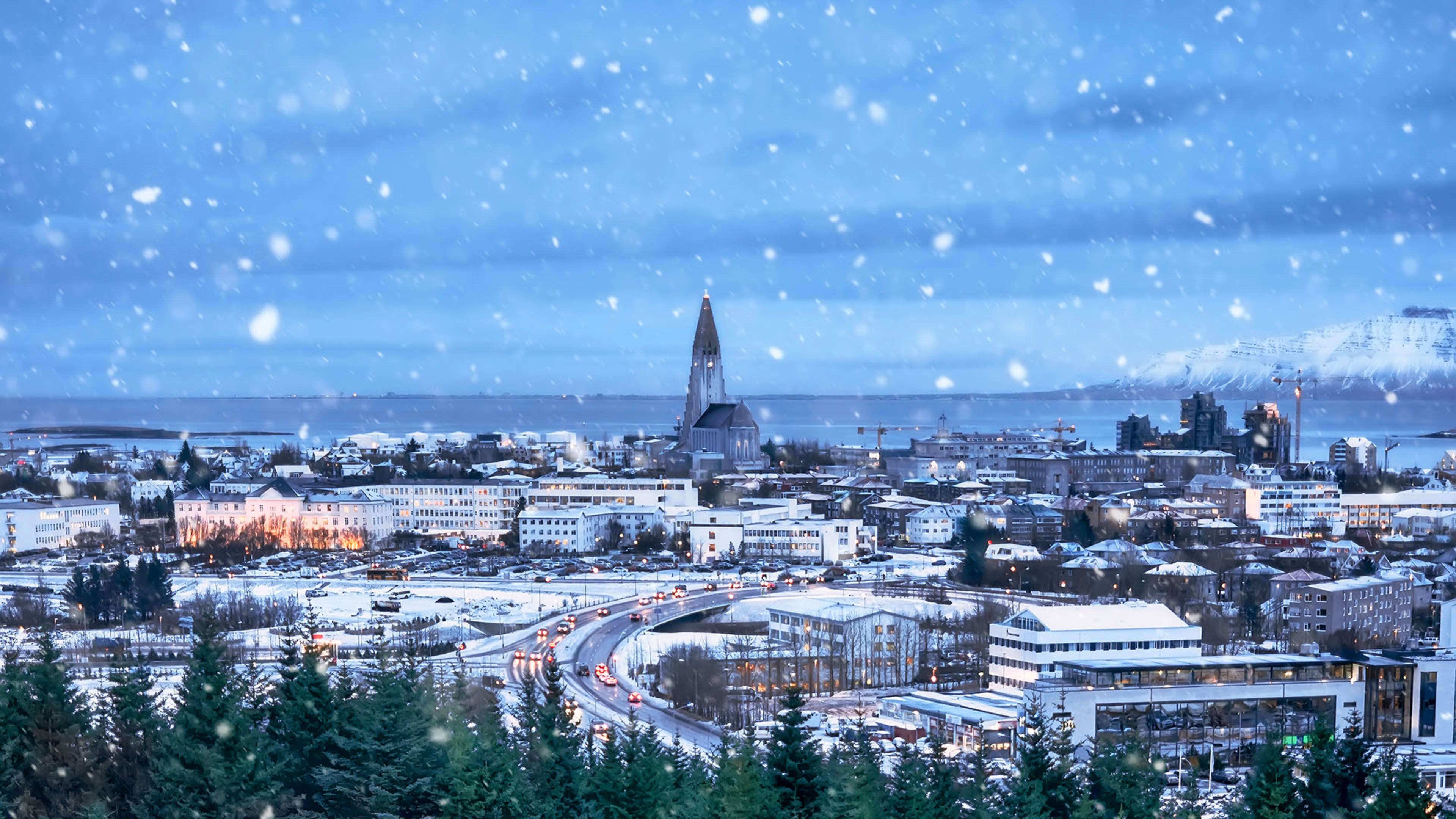This image depicts a picturesque, snowy cityscape by the ocean, seemingly rendered in a postcard style. The scene is set at night, as evidenced by the dark blue sky and the illuminated headlights of cars traversing wet streets. Snow is gently falling, indicated by numerous white dots dotting the sky. 

The city is viewed from an elevated vantage point, possibly a hill, giving a broad overlook. A dominating feature in the center is a tall church with a steeple topped by a gold cross, which stretches impressively into the cloudy, grayish-blue sky. The buildings in the city display varying colors, with the left side showing predominantly white structures and the right side gray ones, all dusted with snow. 

Below the buildings, a couple of four-lane roads are visible, one heading into the city and the other out, lined with cars whose lights glow against the snowy backdrop. Thick pine trees frame the bottom edge of the image, adding to the serene winter atmosphere. In the distance, across a thin strip of water, an island is visible, completely blanketed in snow beneath the right-hand corner dominated by a snow-capped mountain.